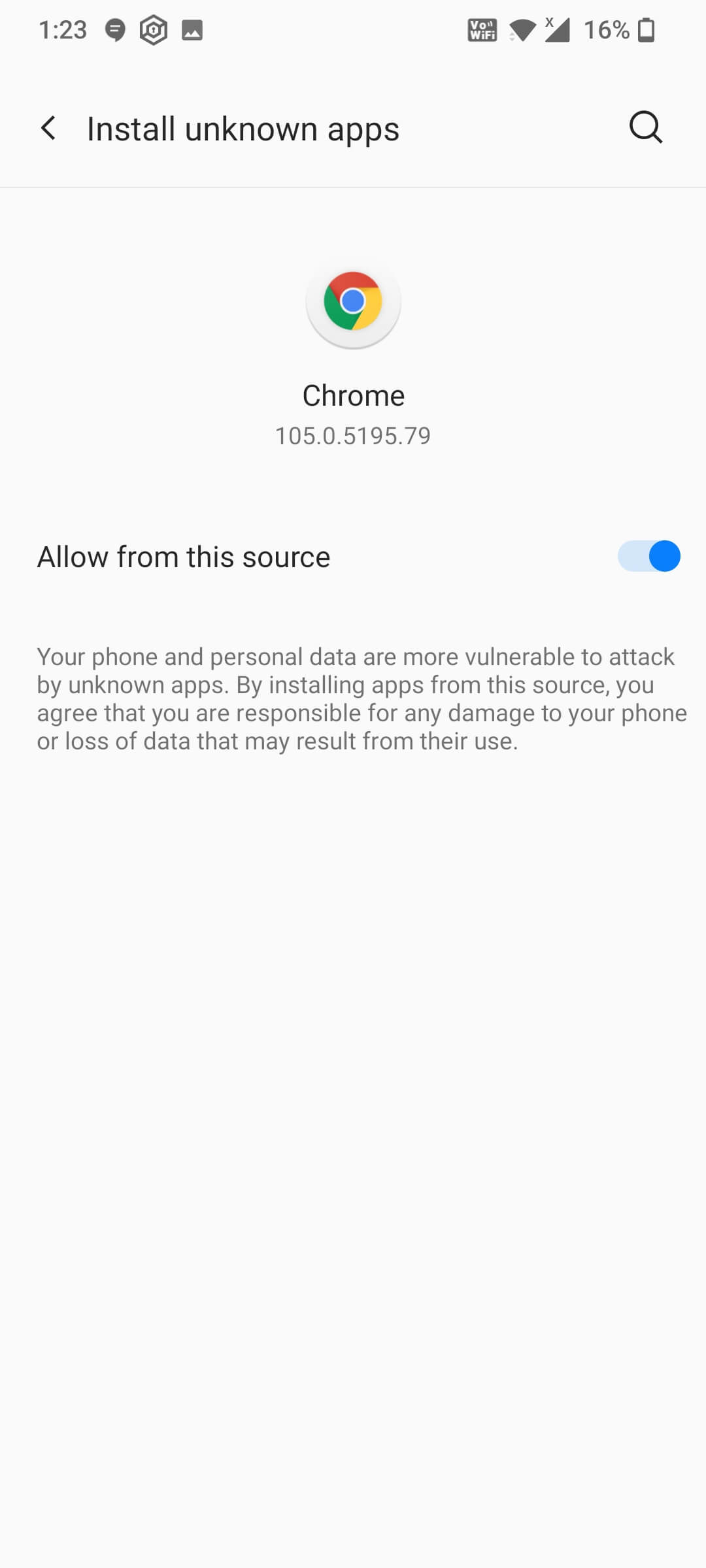This detailed caption describes the image of a smartphone screen displaying settings for app installations:

The image shows a smartphone screen with a page dedicated to app installation settings for Google Chrome. The background of the page is white, and the content is centered towards the top, leaving a significant portion of the lower area blank. At the top of the screen, the status bar indicates that the phone has 16% battery remaining, no cellular signal bars, and low Wi-Fi connectivity.

The heading on the page reads "Install Unknown Apps," accompanied by a magnifying glass icon. Below this, it specifies the app in question as "Chrome," with the version listed as "Chrome 105.0.5193.79." A toggle switch labeled "Allow from this source" is activated, indicated by its blue color. This permits the installation of apps from this source.

A warning message is displayed in black text: "Your phone and personal data are more vulnerable to attack by unknown apps. By installing apps from this source, you agree that you are responsible for any damage to your phone or loss of data that may result from its use." Additionally, the familiar Chrome icon is visible, characterized by a circle divided into red, yellow, and green segments with a blue center.

The overall layout is minimalistic, emphasizing the potential risks of installing apps from unknown sources, as highlighted by the crisp, clear text and the contrasting areas of color and whitespace.